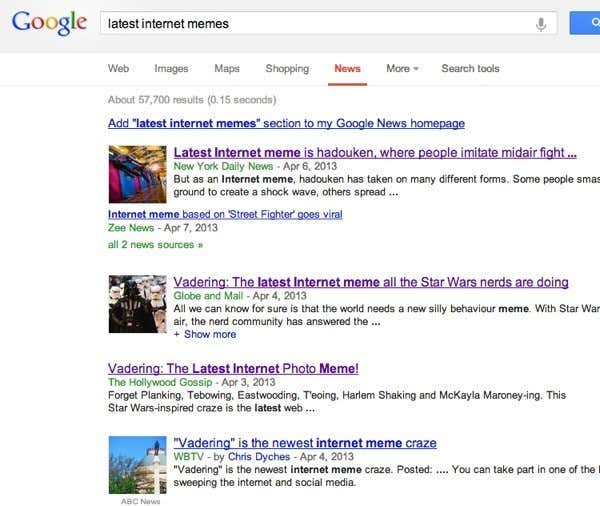This screenshot captures a Google search results page displayed in landscape mode, featuring the query "latest internet memes" typed into the search bar. In the top left corner, Google's distinctive logo is clearly visible. The interface shows tabs labeled 'Web, Images, Maps, Shopping,' with the 'News' tab selected and underlined in red. 

Below the search bar, there is a prompt indicating approximately 57,700 search results. There is a live link suggesting the option, "Add latest internet memes to my Google News homepage."

The search results predominantly focus on internet memes from April 2013. The top search result, marked in purple illustrating a previously visited link, discusses the "HADOUKEN" meme where people imitate midair fighting from the popular game Street Fighter, dated April 7, 2013. Another set of purple links refer to the "Vadering" meme, inspired by the Star Wars character Darth Vader, with entries dated April 3 and 4, 2013.

Additionally, a blue link appears mentioning the "newest internet meme craze," dated April 4, 2013. The repetition of 2013 dates suggests a filter has been applied to show only results from that specific year.

Overall, the live links in the screenshot include: "Add latest internet memes," "latest internet meme," "internet meme based on Street Fighter," and multiple links related to "Vadering." Some portions of the interface, such as a blue button on the upper right, are slightly cut off, hinting that the screenshot only captures part of the webpage.